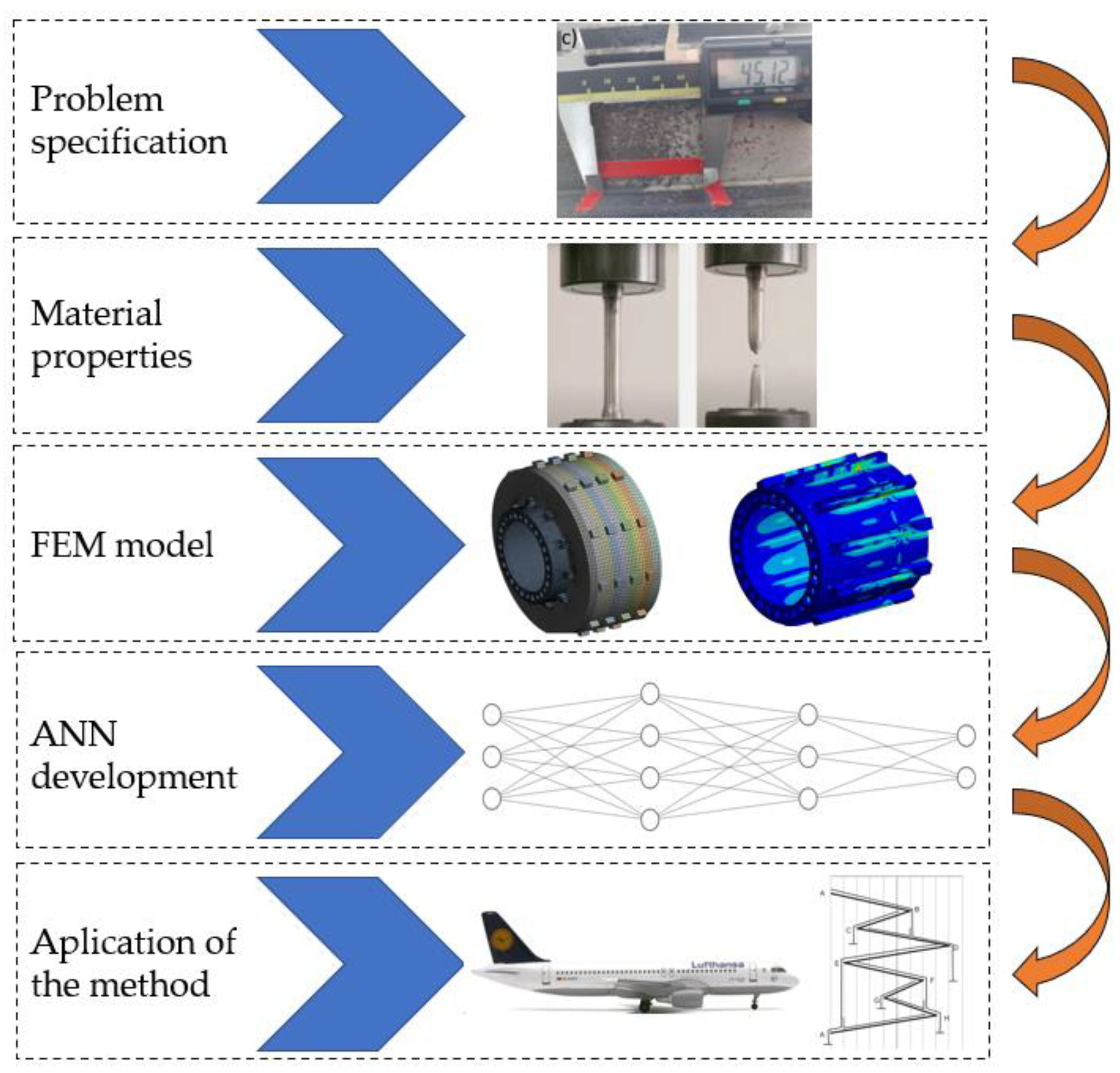This detailed flowchart illustrates the development of an industrial strategy for resolving airplane control issues through five clearly defined stages. The chart is divided into five sequential, rectangular sections stacked vertically, each connected by a prominent blue arrow that guides the flow from top to bottom. 

1. **Problem Specification**: This initial stage features text describing the problem on the left side, followed by a large blue arrow pointing to a picture of measuring equipment with a small digital screen.
2. **Material Properties**: The second section is similarly structured with descriptive text, a blue arrow, and an image showcasing a metal rod attached to a base, indicating the evaluation of material properties.
3. **FEM Model**: The third segment follows with explanatory text, a blue arrow, and an image of circular mechanical parts, likely representing finite element modeling (FEM).
4. **ANN Development**: Next, this section includes descriptive text, a blue arrow, and a chart of interconnected lines and circles illustrating the development of an artificial neural network (ANN).
5. **Application of the Method**: The final section features text summarizing how the method is applied, concluded by a blue arrow leading to a photo of a flying airplane. 

Accompanying the airplane image is a gray jagged line on the right side, representing dynamic changes or flight paths, and an orange arrow looping to connect different parts of the page, emphasizing the iterative nature of the process.

Overall, the flowchart effectively combines text, images, and illustrative diagrams to provide a comprehensive overview of the strategic development process for resolving airplane control issues.